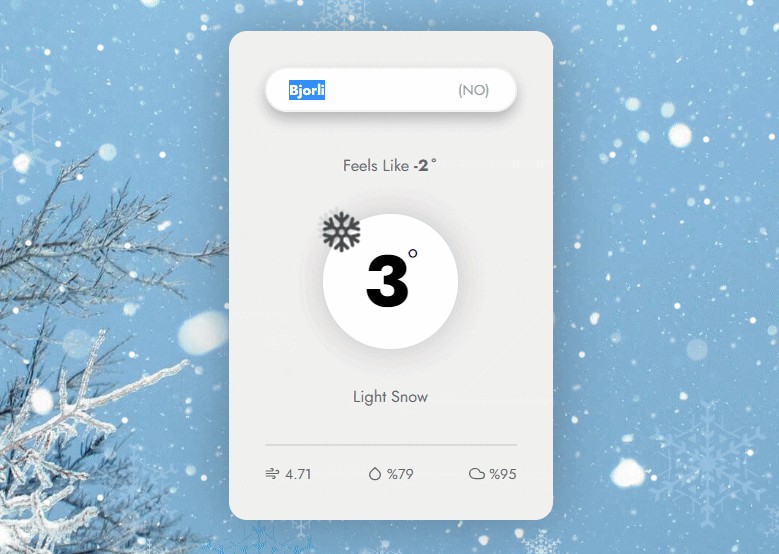The image is in landscape format and rendered in vibrant color. It appears to be a screen capture of a laptop desktop background, solely featuring the generic background without visible taskbar elements. The background illustrates a winter scene, looking skyward through a cascade of falling snowdrops in various sizes, some appearing larger as they pass near the camera lens. The scene is framed by snow-covered coniferous trees rising on the bottom left, enhancing the wintry atmosphere.

Centrally, a window is open, displaying the text "B-J-O-R-L-I," which seems to be highlighted or selected, possibly indicating a copying or pasting action. Below this text, the current weather information is prominently shown: a large printed "3°C" with the note that it "feels like -2°C." The weather is described as "light snow," with additional details showing a wind speed of 4.71 m/s and a 79% chance of precipitation.